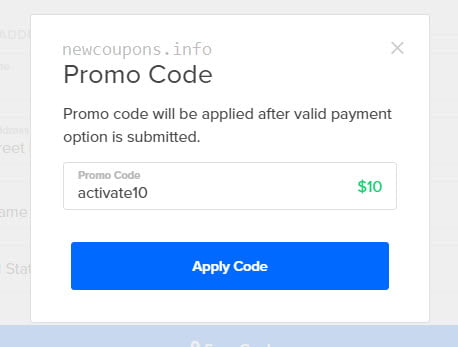The image displays a pop-up promo code on a website, highlighted against a grayed-out background with black text. The promo code section itself stands out with a white background. At the top, "newscoupons.info" is subtly printed in light gray. Beneath this, the bold, black text reading "Promo Code" is the focus. At the upper right corner, there's an "X" button to close the pop-up. Below the main heading, a notice states, "Promo code will be applied after valid payment option is submitted." 

A prominent text box is displayed below, with "Promo Code" inscribed inside of it in light gray. Inside this text box is the actual promo code, "ACTIVATE10," in black text, making it easily noticeable. Adjacent to this, on the right side, the value "$10" is highlighted in green, emphasizing the discount's value.

Directly below the text box, a striking blue button reads "Apply Code" in thick, white letters, ensuring it stands out clearly for the user to take action.